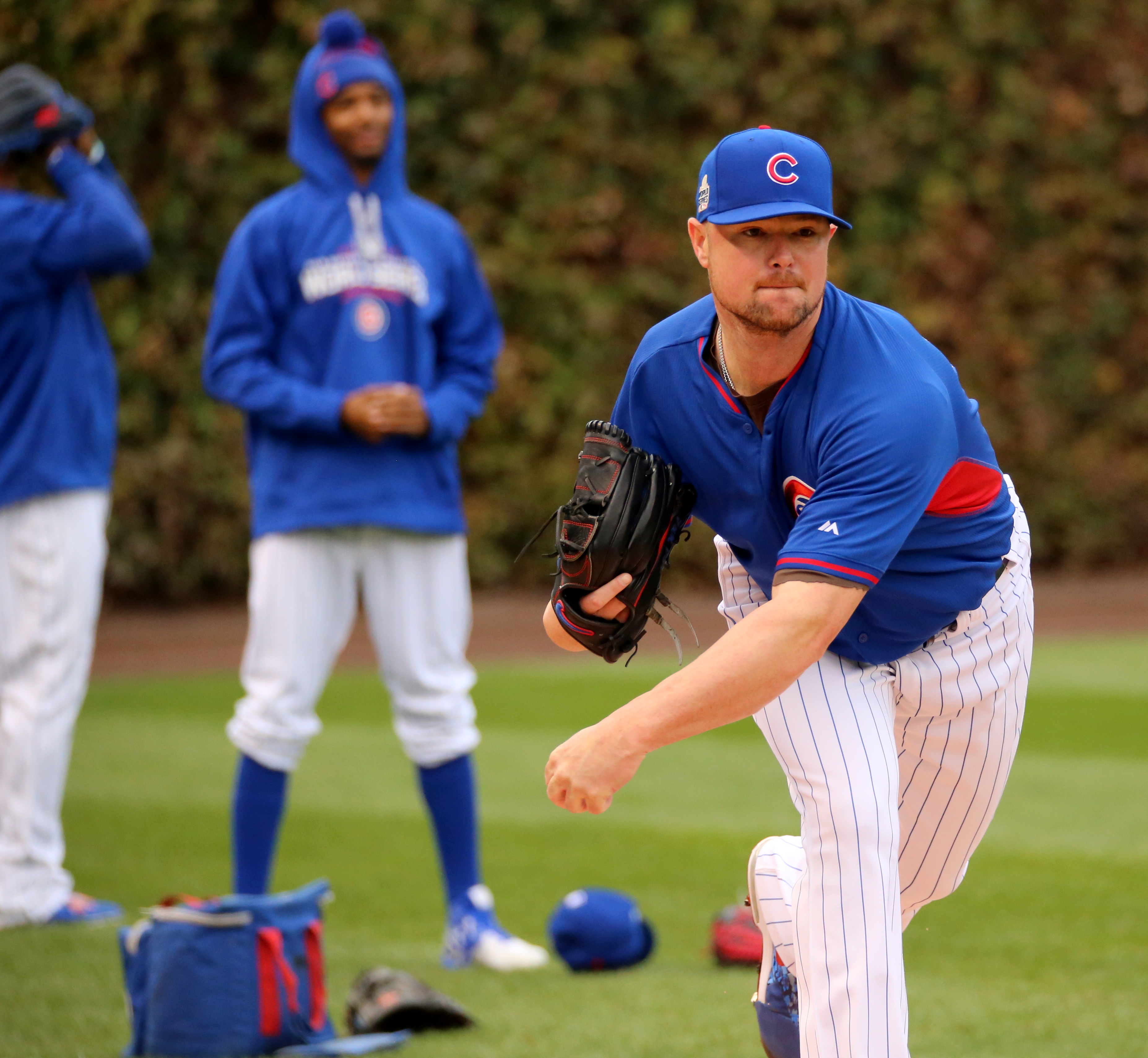The image depicts a professional baseball player just right of center, captured in mid-pitch. He is dressed in a complete game day uniform consisting of a blue cap with a red "C," a blue jersey with red accents, and white pants with vertical blue or black stripes. His attire also includes blue socks and a black and red glove. He has a reddish skin tone, a black beard, and appears to be in his 30s, focusing intently on his pitch. In the background, slightly out of focus, are two other players. One is an African-American man wearing a similar uniform but with a hoodie, and the other has a blue cap adorned with a red and white "C." Both figures seem to be observing the practice. The setting is a baseball field with visible green grass, dirt, and various equipment on the ground, including helmets, a bag, and a glove. Behind the players is a vine-covered wall, adding a touch of greenery to the scene. This professional shot emphasizes the concentration and atmosphere of a baseball practice session.